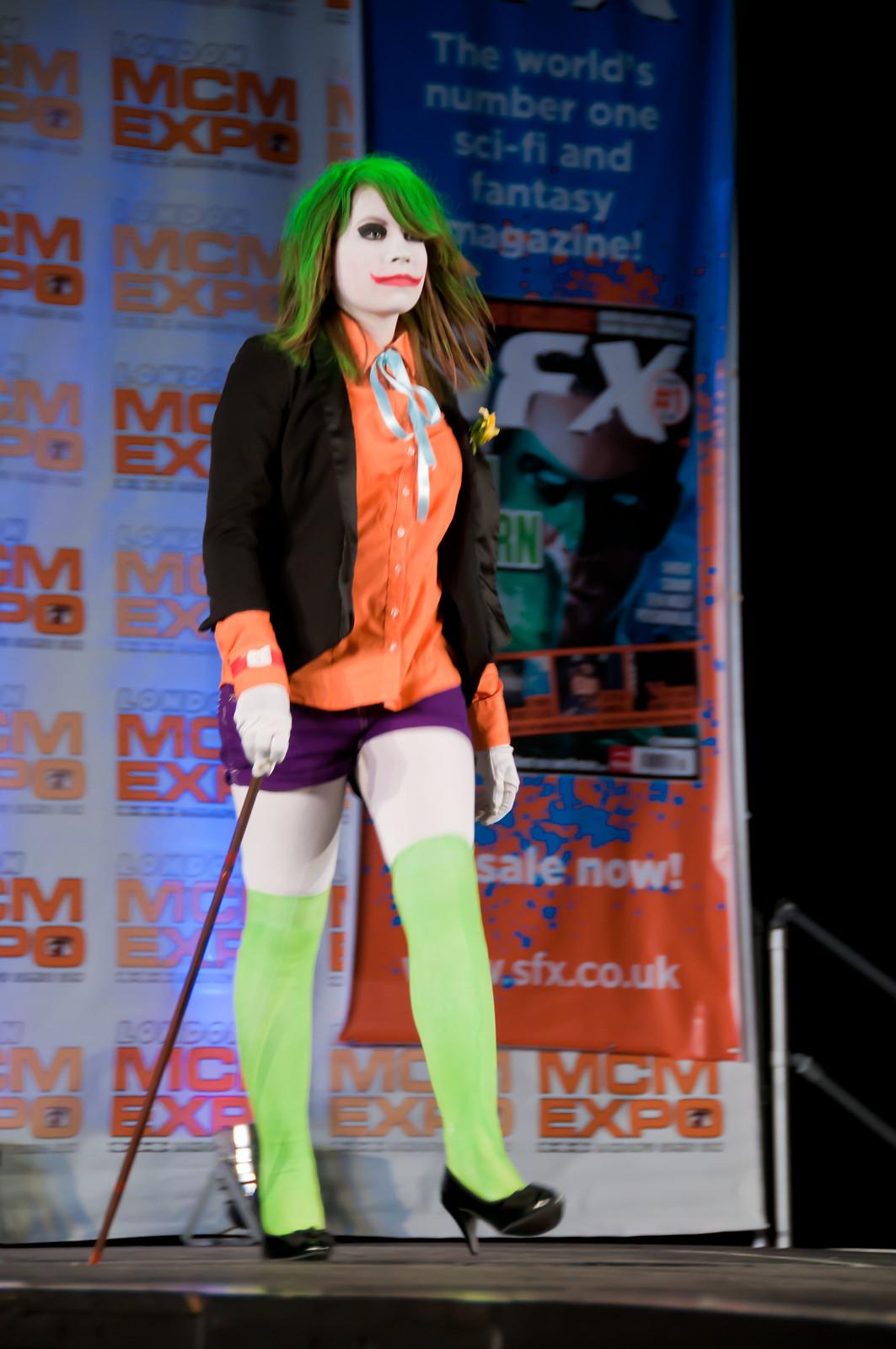At a bustling MCM Expo, in front of a banner declaring “the world’s number one sci-fi and fantasy magazine, SFX, on sale now," an individual strides confidently across a catwalk, decked out in a meticulous female version of the Joker cosplay. She has long, vibrant green hair cascading down her back and is adorned in striking white face makeup and iconic red Joker lips. Her costume includes a salmon pink button-up shirt with a silver ribbon tie, a black suit jacket featuring a small yellow flower, and red shorts. Enhancing the look, she wears bright lime green stockings pulled up just over the knees, paired with black high-heeled shoes. She completes her ensemble with a purple cane held in her right hand and white gloves. The detailed makeup and elaborate outfit make her a vibrant focal point against the backdrop of the sci-fi and fantasy-themed event.